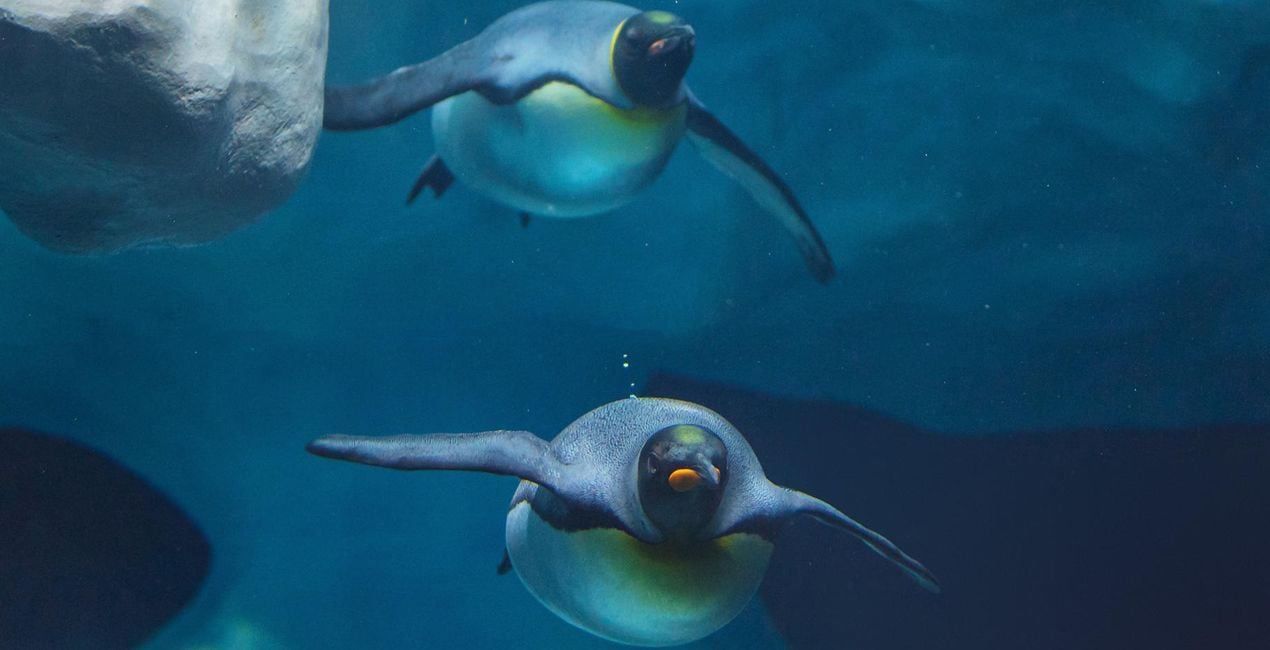In this underwater photograph, two penguins glide gracefully through the water, their rotund bodies creating a captivating scene. Positioned respectively near the top and bottom of the image, these penguins are depicted with black upper bodies and white lower bodies, complemented by a subtle yellow patch beneath their beaks. One penguin features an orange beak while the other has a black beak. The vibrant blue water envelops them, with the background predominantly a soothing dark blue, evoking a serene underwater environment. The penguins' black flippers extend parallel to the ground, accentuating their streamlined shape. In the top left corner, a gray rock juts out, adding a touch of rugged texture to the soft fluidity of the image. This scene could either be a real glimpse into a natural underwater habitat or a meticulously crafted aquarium display, as the penguins possess an almost lifelike yet slightly artificial appearance.